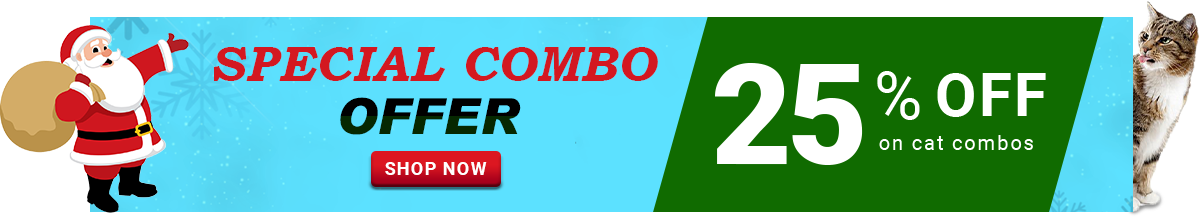The image features a pristine white background adorned with a subtle pattern of snowflakes. Dominating the central space, there’s a vibrant blue and light blue advertisement, evoking a wintry feel. On the right side of the ad, there’s a dark green box with diagonally cut sides. Inside the box, bold white text prominently displays "25%" with smaller capital letters spelling "OFF" beneath it. In tiny lowercase letters below that, the text reads "Cat Combos."

To the left of this box, an illustration of Santa Claus catches the eye, depicted with his bag slung over one shoulder and his other arm raised cheerfully. Just in front of Santa, the words "Special Combo" are emblazoned in large red capital letters. Directly below this, the word "Offer" is presented in black capital letters. At the bottom of this section, there is a bright red button that invites viewers to "Shop Now."

On the right side of the image, a gray tabby cat with a white chest is shown gazing towards Santa Claus and the enticing offer, adding a touch of festive whimsy to the scene.